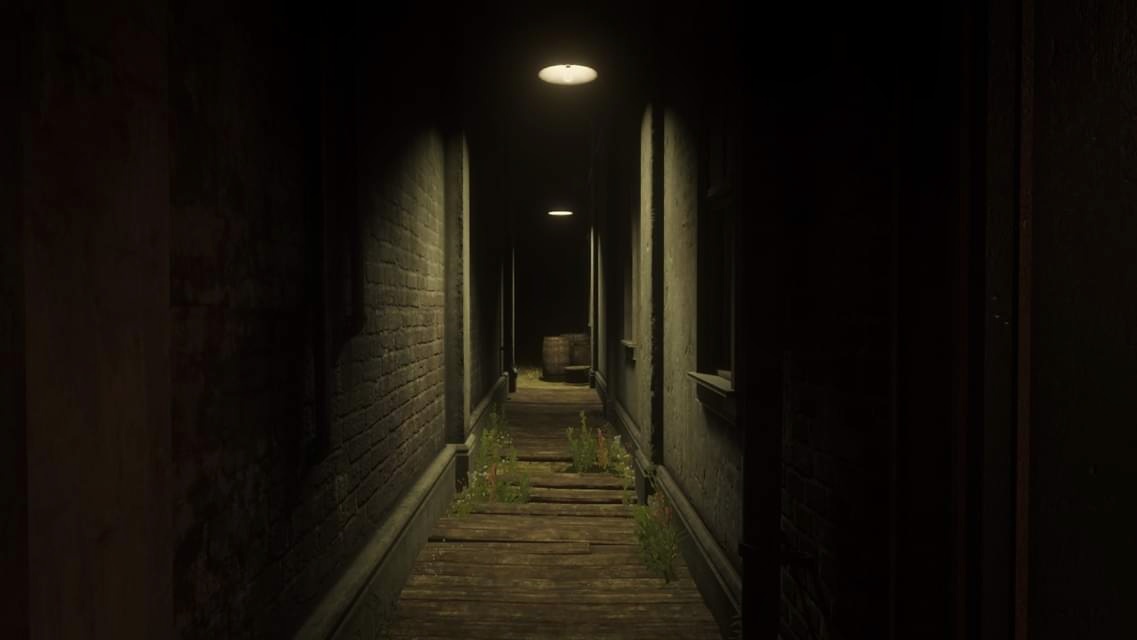This photograph captures an extremely dark alleyway or narrow hallway framed between two buildings. The left building features a dirty brick facade that appears brown due to aged grime, while the right building sports a smooth, gray stucco surface. The ground is covered by old wooden planks laid perpendicularly, which resemble railroad ties, with tufts of grass and weeds growing through the gaps. The only illumination comes from two meager overhead lights, casting faint white beams along the walkway. Further down the corridor, two small brown barrels can be seen amid the shadows, with one positioned more centrally and the other slightly to the right, beside what looks like a small step. The lack of substantial lighting and the encroaching darkness make this space unwelcoming.